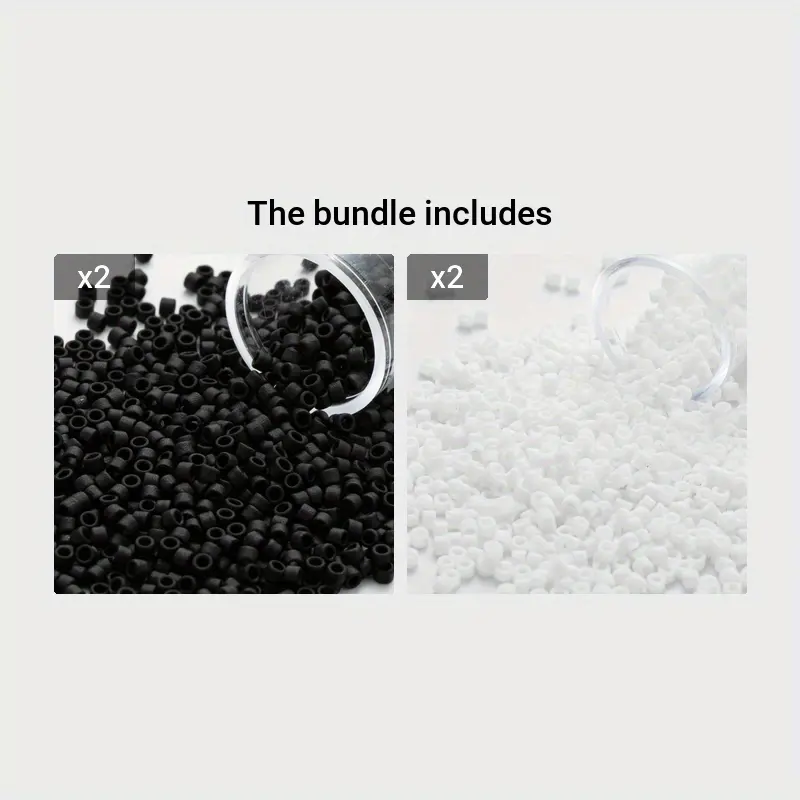The image features two black and white photographs set against a pale gray background, both labeled with the text "The Bundle Includes" at the top. Each photograph displays the same label, "X2," indicating that the items are multiplied by two. On the left, a clear glass jar, positioned at the top right of the photo, is pouring out numerous small, black seed beads or plastic pellets. This photograph captures the details clearly, showing the beads scattered across the surface. On the right, an overexposed photograph depicts a similar clear glass jar pouring out small, white plastic beads or pellets. Due to the overexposure, the details of the white beads are much harder to discern, but the juxtaposition with the left-hand image makes it evident that they are the same type of objects in a different color. Both images suggest the beads are likely used for crafting purposes, like making beaded necklaces or bracelets.